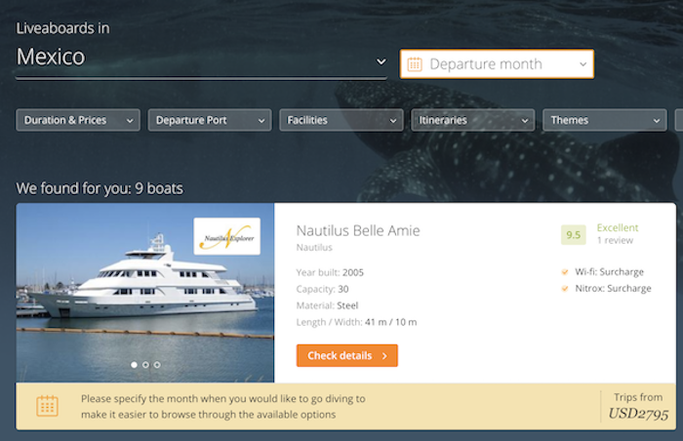In this horizontally oriented screenshot, set against a predominantly black background interspersed with shades of gray, you can discern a very darkened image of a shark swimming in the lower right corner. The upper left corner displays the text "Liveaboards in Mexico" in light gray. In the upper right corner, there's a pull-down menu labeled "Departure Month," accompanied by a calendar icon. Adjacent to this, from left to right, are various filters in gray text: "Duration and Prices," "Departure Port," "Facilities," "Itineraries," and "Themes." The search results indicate, "We found for you nine boats." The first boat listed is a large yacht named Nautilus Belle Amie, built in 2005, with a capacity of 30 people and constructed of steel. In the lower right corner, there's a review rating of 9.5, labeled as "Excellent," from a single review.